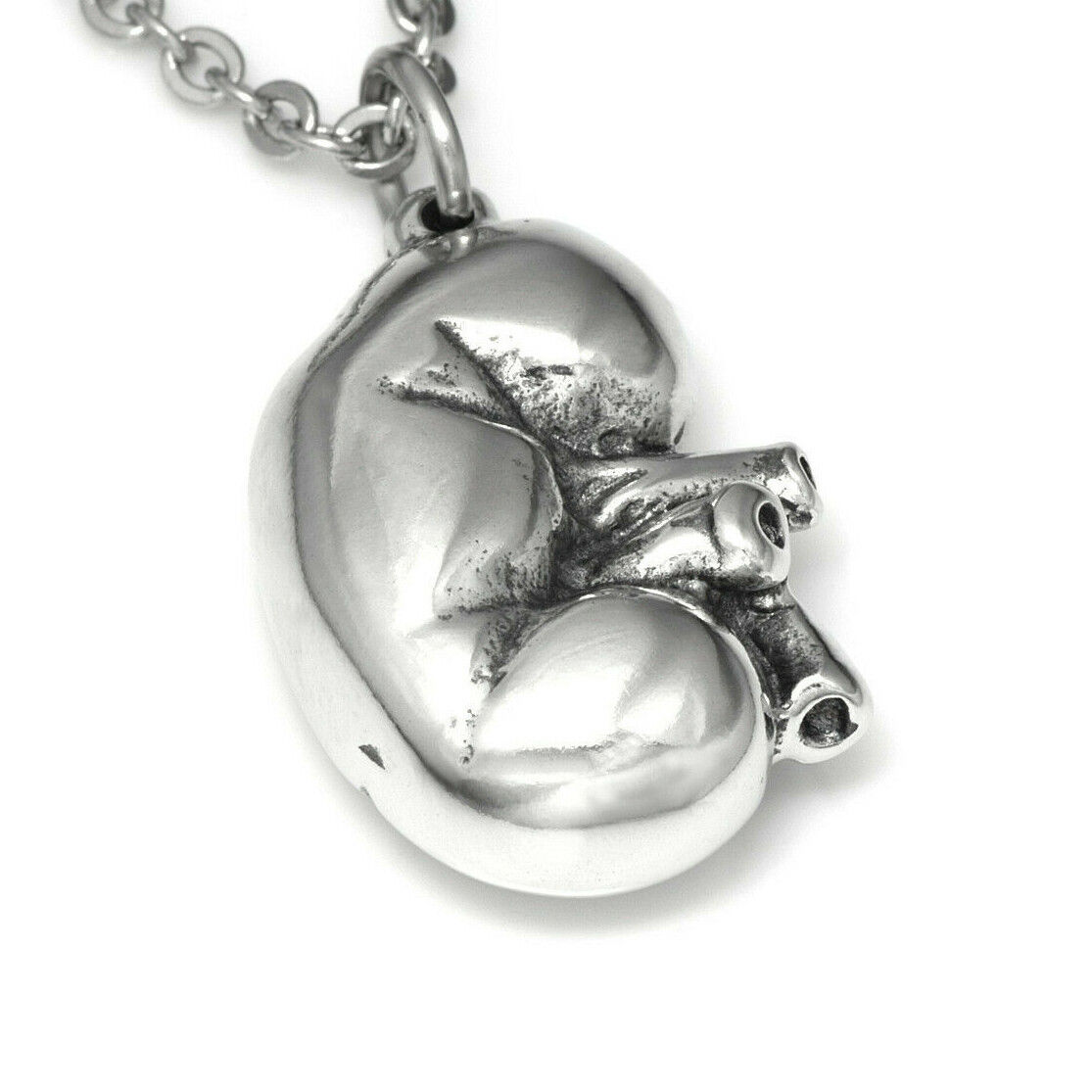In this professional close-up image designed for online sale, a silver necklace is prominently displayed against a white background. The main focus is the pendant, hanging diagonally to the left, and it resembles an anatomical heart, complete with various protruding vessels and valves. Despite its heart-like qualities, the pendant also evokes the shape of a kidney bean with arteries emerging from it. The highly polished silver surface of both the pendant and the partially visible chain reflects the camera's flash, adding a shiny, reflective quality to the piece. The chain, extending toward the upper left of the image, reveals about six links connected to a ring at the top of the pendant. There is no text or additional background elements, ensuring that the intricate details of the jewelry are the sole focus of the photograph.